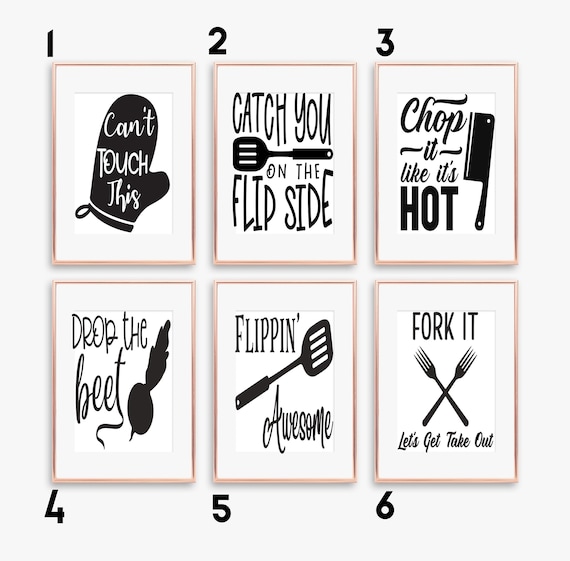This image features six framed prints, arranged in two rows of three, that bring a humorous touch to kitchen decor. Each print is set against a white background with black illustrations and text, bordered by a pinkish-beige frame. The prints are labeled from one to six, each showcasing a witty kitchen-related phrase along with a relevant utensil:

1. "Can't Touch This" - Depicts a black oven mitt.
2. "Catch You on the Flip Side" - Features a black spatula.
3. "Chop It Like It's Hot" - Shows a black meat cleaver.
4. "Drop the Beet" - Illustrates a black outline of a beet vegetable.
5. "Flippin' Awesome" - Displays another black spatula.
6. "Fork It, Let's Get Takeout" - Includes two black forks crossed in an X-shape.

The prints suggest a playful approach to cooking and kitchen tasks, reminiscent of items that might be found on Etsy or in a trendy home decor store.